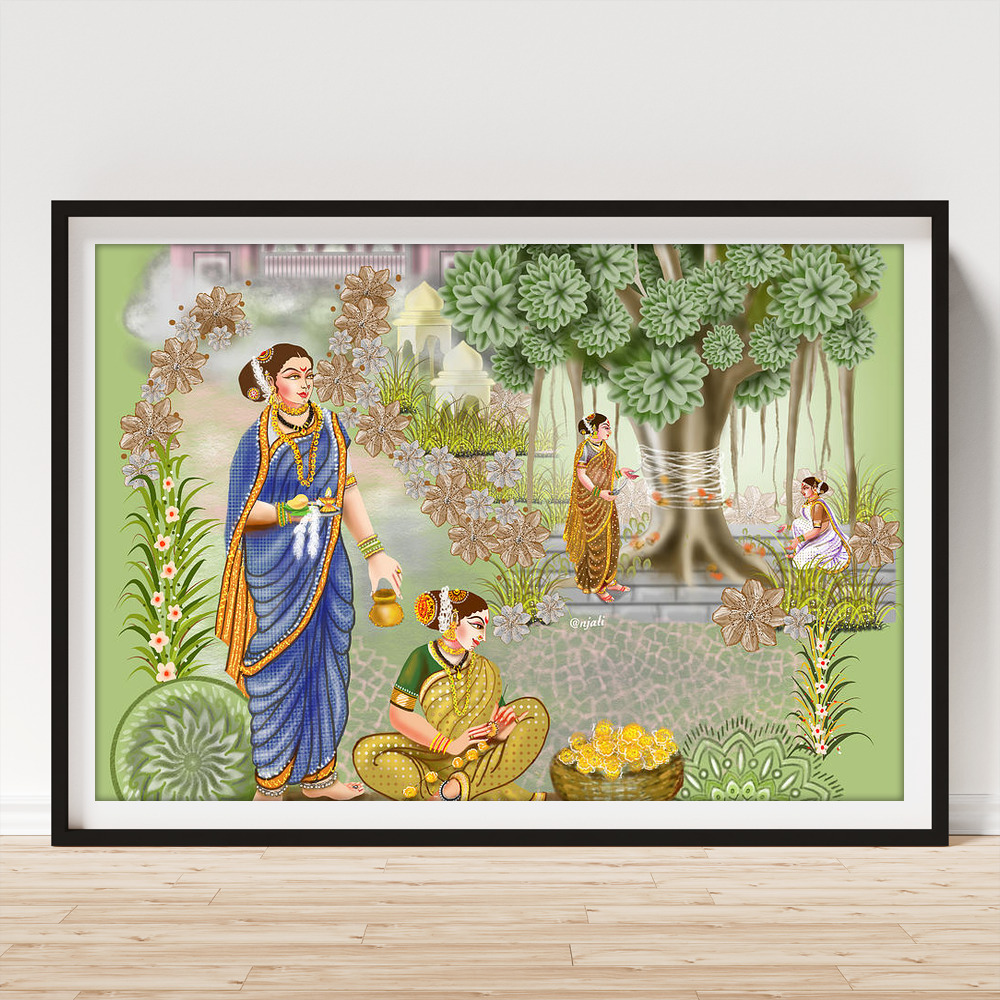The artwork is a large, intricately detailed painting leaning against a stark white wall, framed by a thin black border and a wide white mat. It rests on a light brown, wood plank floor. The main scene depicts four Indian women adorned in traditional saris, richly decorated with gold accents, jewelry, and flowers in their hair, evoking a sense of elegance and historical charm.

In the foreground, a woman dressed in a blue sari stands gracefully. She holds a small golden flask in one hand and a collection of feathers in the other. Below her, another woman, clothed in an olive green sari, sits cross-legged on the ground with a large basket of vibrant yellow flowers in front of her. She seems to be weaving or sewing the flowers into a garland or bracelet.

Towards the background, to the right side of the painting, a large tree takes prominence. Two women are positioned around the tree; one is standing, adorned in a gold dress and facing a palace or temple drawn in the distant backdrop, while the other kneels on the ground, engaged with what appears to be string or twine wrapped around the tree, with apples falling around them and flowers incorporated into the design. The overall scene is set in a lush garden with an abundance of greenery, blues, and golds, framing the tranquil and timeless moment captured in the painting.